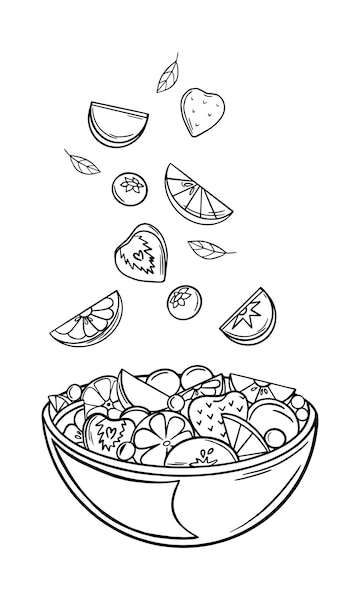This detailed line art illustration, rendered entirely in black and white, showcases an assortment of fruit pieces both in and above a uniquely shaped bowl. The art is done with clean, precise pen lines, giving it a crisp, clean appearance typical of a well-executed ink drawing. 

The bowl, which appears to be half a bowl or a bowl bisected, already contains various fruit pieces such as lemon wedges, strawberries, and blueberries. Suspended above the bowl, more fruit pieces, including strawberries with small leaves, citrus sections, and additional leaves, appear to be falling into it, creating a dynamic sense of motion. 

The overall contrast between the black outlines and the white interior of the drawing accentuates the different types of fruit, despite their monochromatic representation. This striking illustration combines clarity and simplicity to depict a lively scene of a fruit bowl being filled. The bowl itself is mainly white with distinct black lines outlining its form, enhancing the distinct line art style of the illustration.